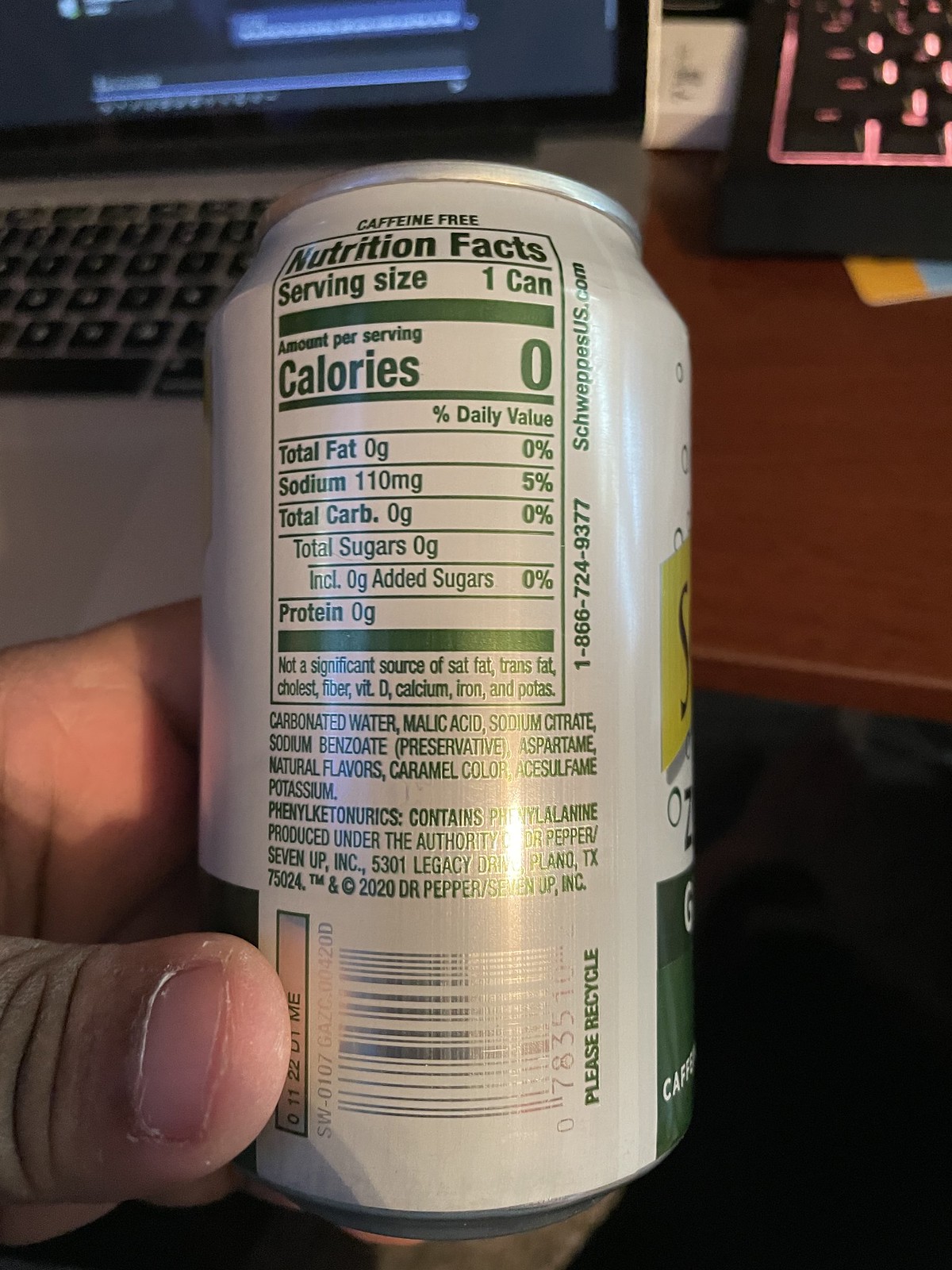The image depicts a white aluminum soda can with green writing, prominently displaying nutrition facts on its rear side. The can is labeled "caffeine-free" and detailed with a green outline. Specific nutritional information includes a serving size of one can, zero calories, zero fats, 110 milligrams of sodium, zero carbohydrates, zero sugars (including added sugars), and zero proteins. The ingredients list highlights carbonated water, natural flavors, malic acid, sodium citrate, sodium benzoate as a preservative, aspartame, and caramel color, among others. The can is held by a person, their thumb and part of their palm visible, revealing the nutrition facts to the camera. In the background, a portion of a gray keyboard, part of a laptop screen, and a wooden desk are slightly visible. A hint of the can’s front, featuring an S-shaped letter on an angled yellow background, and a green and yellow label, suggests it might be of a brand like Schweppes.